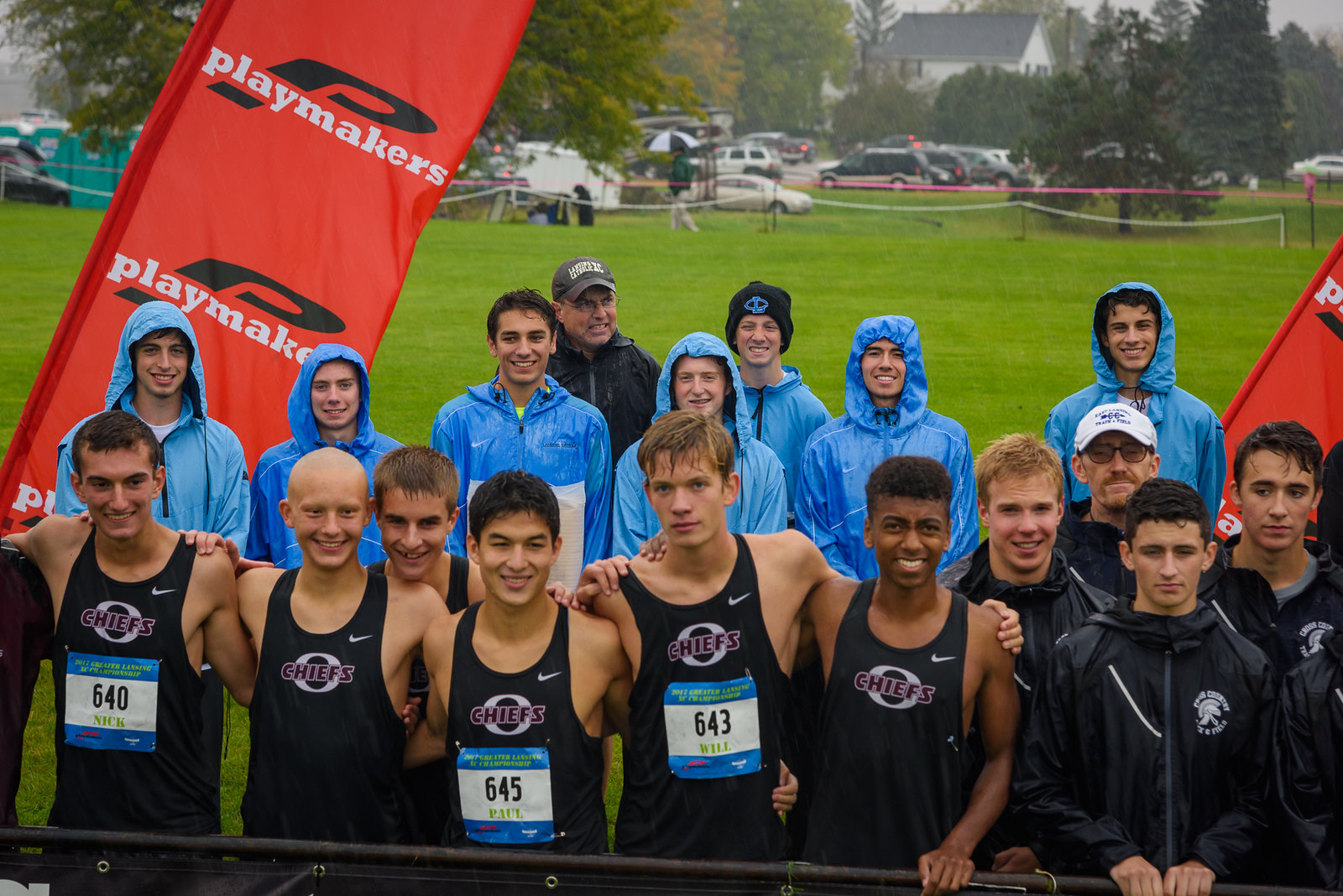This image is a detailed, photorealistic photograph of a male sports team, likely a track or cross-country team, posing outdoors. The front row comprises young boys dressed in black tank tops, each adorned with a white Nike swoosh on the right side and a central logo featuring a white ‘O’ with the word ‘CHEAPS’ in purple. Some members of this front row also wear blue and white race cards with numbers on their tank tops. The second row of boys stands behind them, dressed in blue raincoats or windbreakers, some with their hoods up. At the very back is an older man, possibly the coach, donning a black coat and a brown hat. To the right, partially obscured by the photo's edge, and to the left, a red banner with a black 'P' and ‘PLAYMAKERS’ in white font is firmly planted into the ground.

The setting is a large green grassy field, likely a park or sports field, with trees, parked cars, and house rooftops visible in the distance. Despite the rainy weather indicated by the raincoats, the team gathers closely, exuding a sense of unity as they either prepare for or have just completed a race.